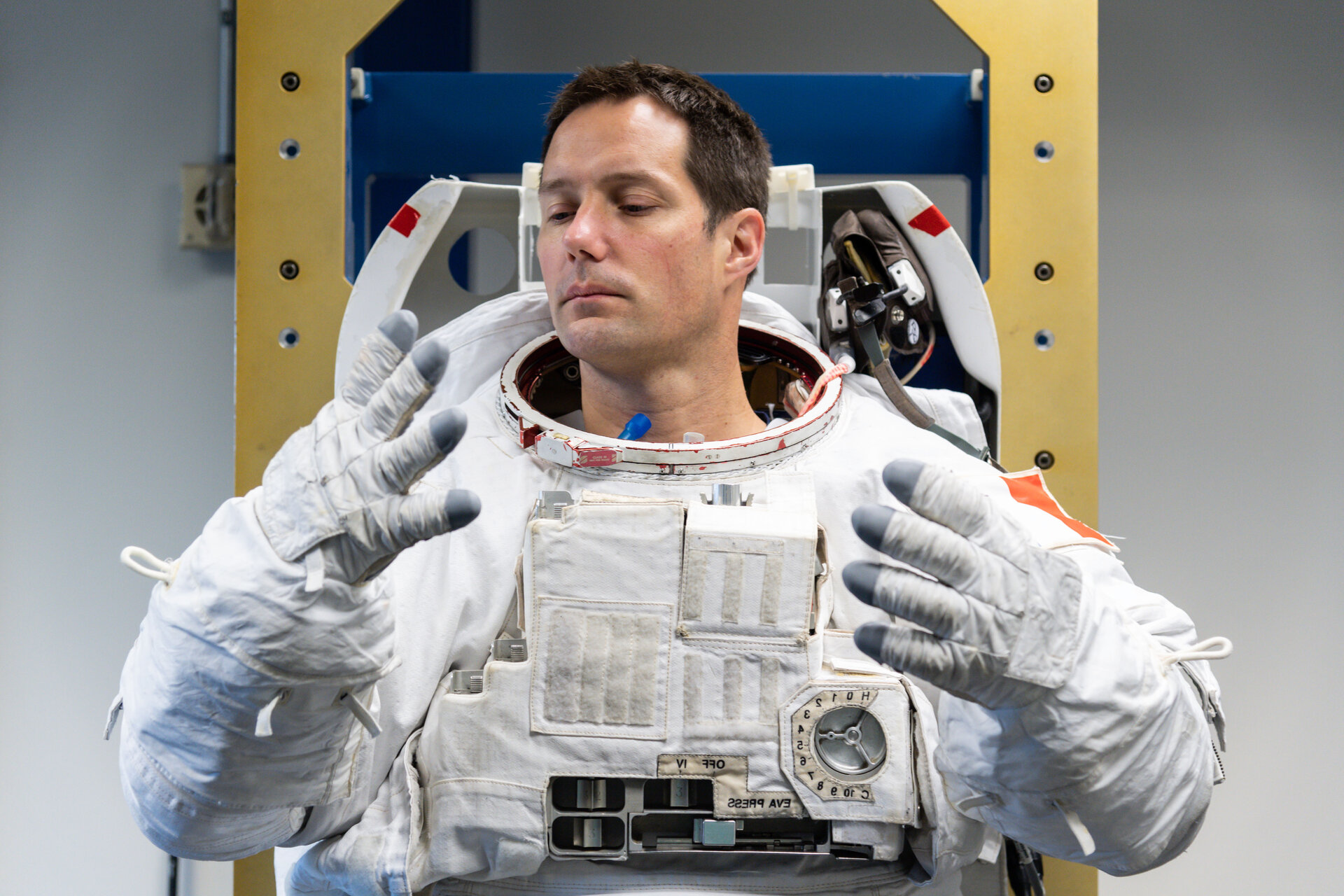The image features a Caucasian man in his mid-thirties with short brown hair, dressed in a full white astronaut suit, complete with thick gloves characterized by gray rubber or silver tips and numerous Velcro fastenings. The suit also has various levers, gauges, and buttons, including a prominent pressure gauge on the front, suggesting functionality for controlling and monitoring life-supporting systems. Notably, he is missing the helmet, revealing his intent gaze downward at his hands, indicating he might be deeply examining the intricacies of his gloves. A significant oxygen pack is affixed to his back. He is positioned against a yellow and blue metal rack with a gray wall in the backdrop, and the white chair he sits in adds to the technical and composed atmosphere. The overall scene captures a moment of scrutinized focus, whether he is an astronaut or someone acquainting himself with the space suit for the first time.